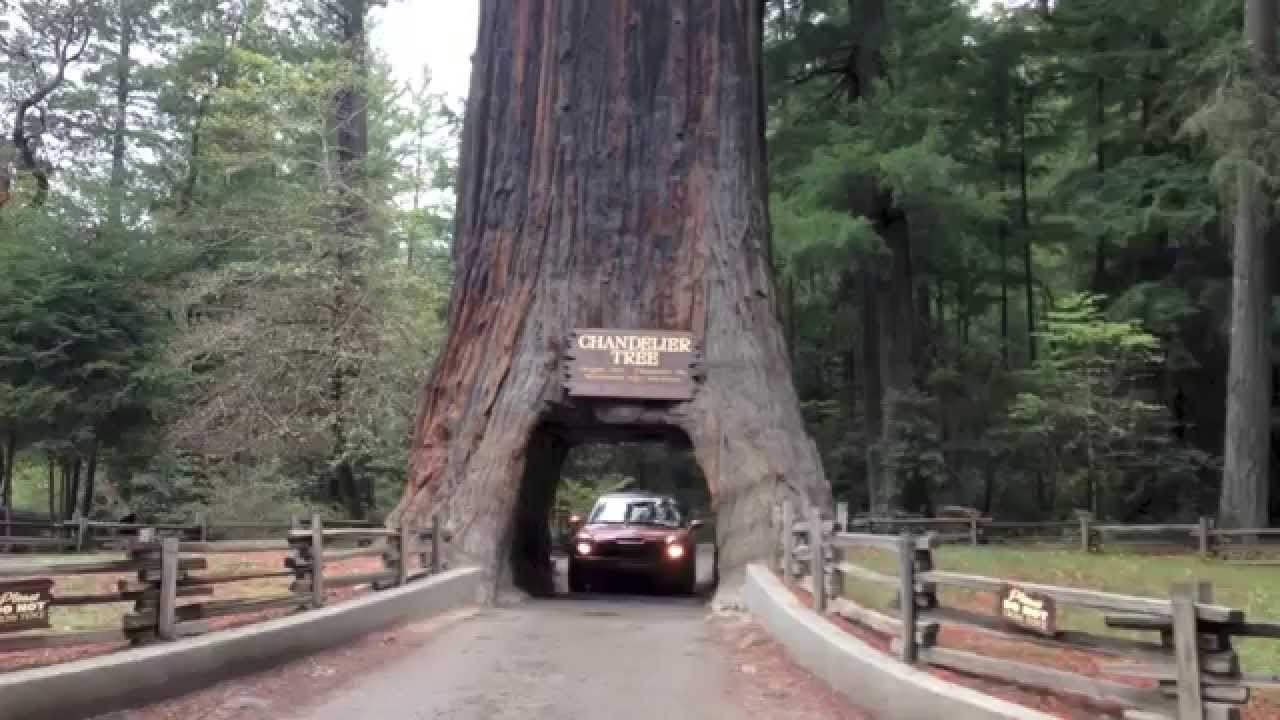The image depicts the renowned Chandelier Tree, a colossal redwood notable for its hollowed trunk that creates a tunnel-like passage through which vehicles can drive. A red car, with its headlights on, is seen traveling through this impressive natural arch. The road is flanked by a combination of short concrete curbs and wooden fences on both sides, ensuring safety and preserving the structure. Surrounding the Chandelier Tree, the forest scene is rich with healthy, verdant trees, showcasing lush greenery and vibrant, healthy leaves that frame the entire backdrop. The massive tree exhibits a unique bark texture, comprising grey, dark, and red tones that accentuate its grandeur. A clearly visible plaque on the tree identifies it as the Chandelier Tree, solidifying its status as a celebrated and significant natural landmark.